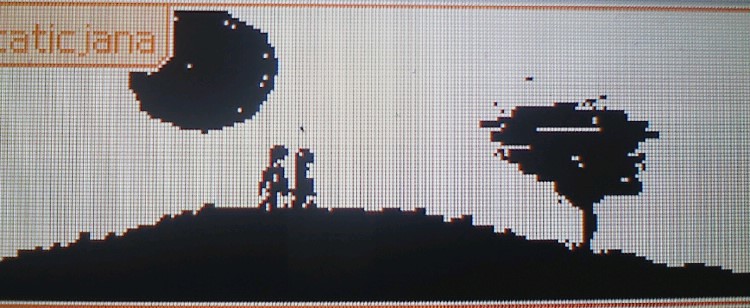The image depicts a screenshot from a very early video game, likely displayed on a portable device from the early era of gaming. The graphics are primitive, with extremely crude, jagged pixels that evoke a sense of nostalgia. On the screen, there are figures—potentially a human and a creature—traversing the serrated edges of a mountain or hill. 

In the backdrop, a pixelated moon with scattered dots and spots enhances the vintage atmosphere. To the right, a menacing figure resembling a monster invader stands with narrow legs and a large torso, hinting at what may be rudimentary gun turrets. The text in the upper left corner reads partially as "A-T-I-C," underlined in a sequence that further spells out "I-A-N-A," rendered in a gray color with a crosshatch pattern.

This scene, with its walkers on a mountainous terrain and coarse, roughly-defined display, encapsulates the essence of early video game graphics, marked by significant limitations in pixelation and design.